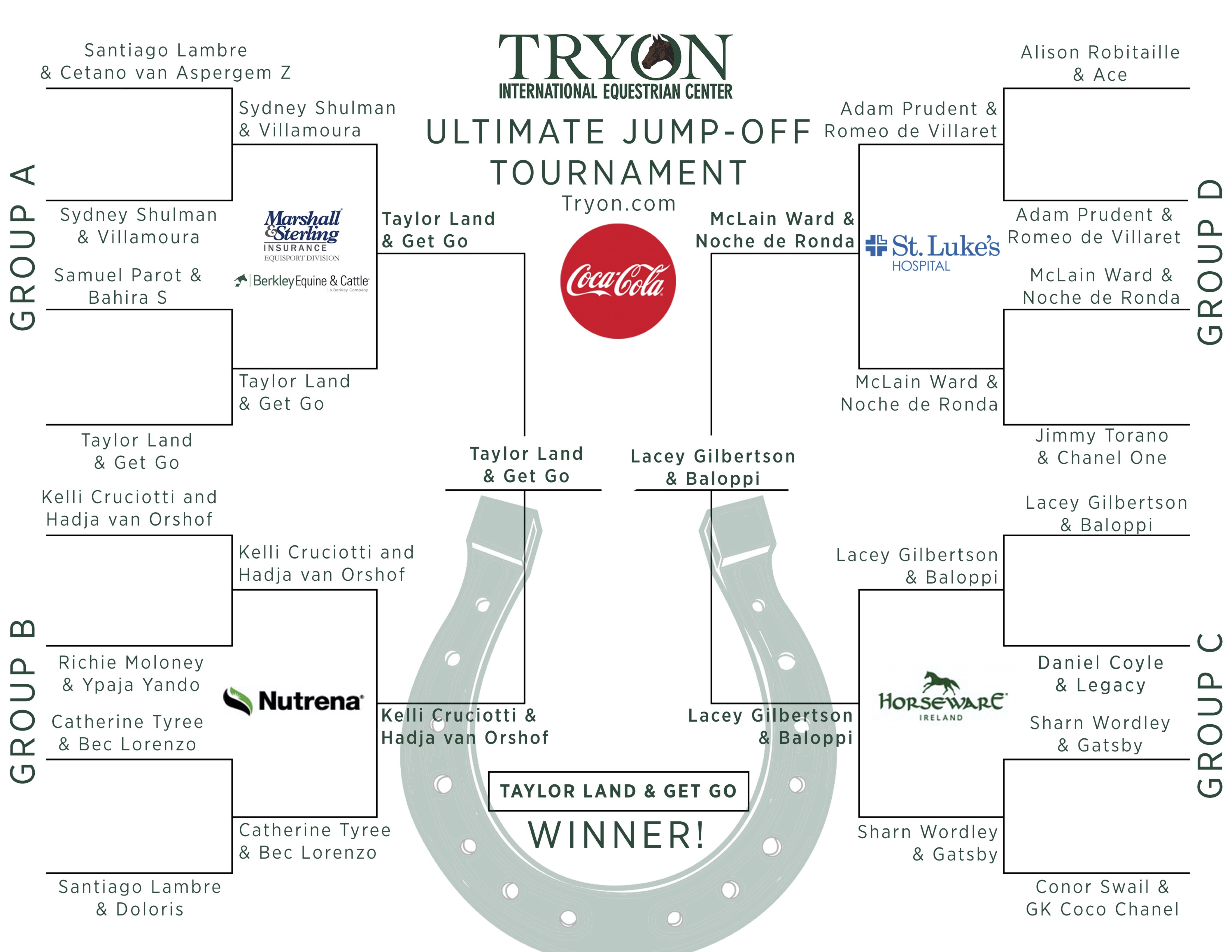The image depicts a detailed tournament bracket from the Tryon International Equestrian Center Ultimate Jump-Off Tournament, set against a white background. At the top of the page, the text "Tryon International Equestrian Center" appears in green, with a stylized horse’s head embedded in the "O" of "Tryon." The bracket illustrates the progress of competitors through four different groups (A, B, C, and D), each vying in an elimination style until only one team remained. The greyish-black horseshoe graphic subtly overlays the background, framed by the prominent red and white Coca-Cola logo centered above. Various sponsors include Coca-Cola, St. Luke's Hospital, Horsewear, Neutrina, and Marshall & Steinberg Insurance. The final competition came down to Taylor Land riding Gitgo versus Lacey Gilbertson riding Biloppi, with Taylor Land and Gitgo emerging as the ultimate victors.